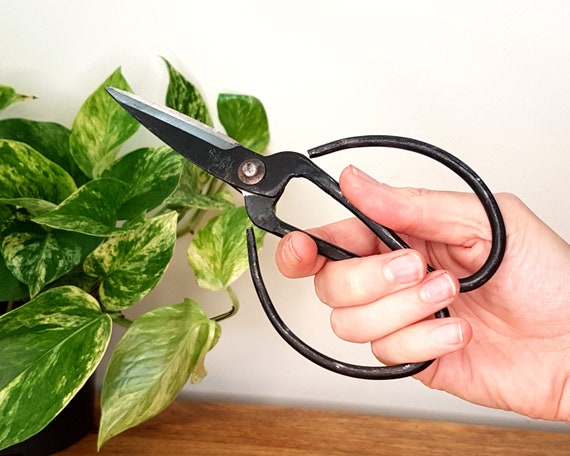The photograph, in full color and horizontally oriented, captures a white hand emerging from the right, gripping a pair of distinctive gardening scissors. These pruning shears feature round, black, all-metal handles and sharp blades, designed to look almost heart-shaped. The hand is positioned with the front facing the camera. To the left, vibrant green and yellow leaves of a philodendron plant extend into the frame, sitting atop a brown wood-stained table. The setting suggests the person is poised to trim the plant, with the backdrop fading into a simple white wall.